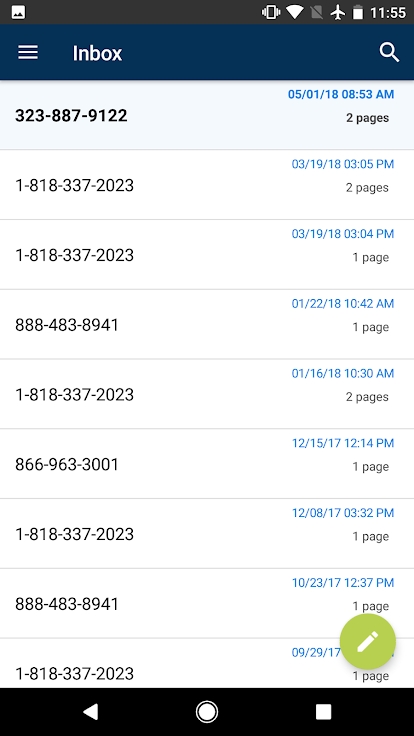This image is a detailed screenshot of an Android device. Located in the top left corner of the status bar is a photo icon. The top right corner displays various status icons, including the vibrate icon, Wi-Fi signal strength indicator, no SIM card icon, flight mode icon, battery level indicator, and the current time, which reads 11:55.

In the main section of the screenshot, there are several phone numbers listed along with the number of associated pages for each entry. The first phone number is 323-887-9122, linked to two pages. The second number is 1-818-337-023, also associated with two pages. A repetition of this second number, 1-818-337-023, is seen again, but this time it is linked to just one page. The following number, 888-483-89411, leads to one page. Another entry, 1-818-337-2023, is connected to two pages. Additionally, there are four more phone numbers listed, though they are not explicitly mentioned in the provided description.

At the bottom of the screenshot, the standard Android navigation keys are visible, which include the back button, home button, and recent apps button. The overall layout suggests that this screenshot might be from a call log or messaging app, displaying various contacts and their details.